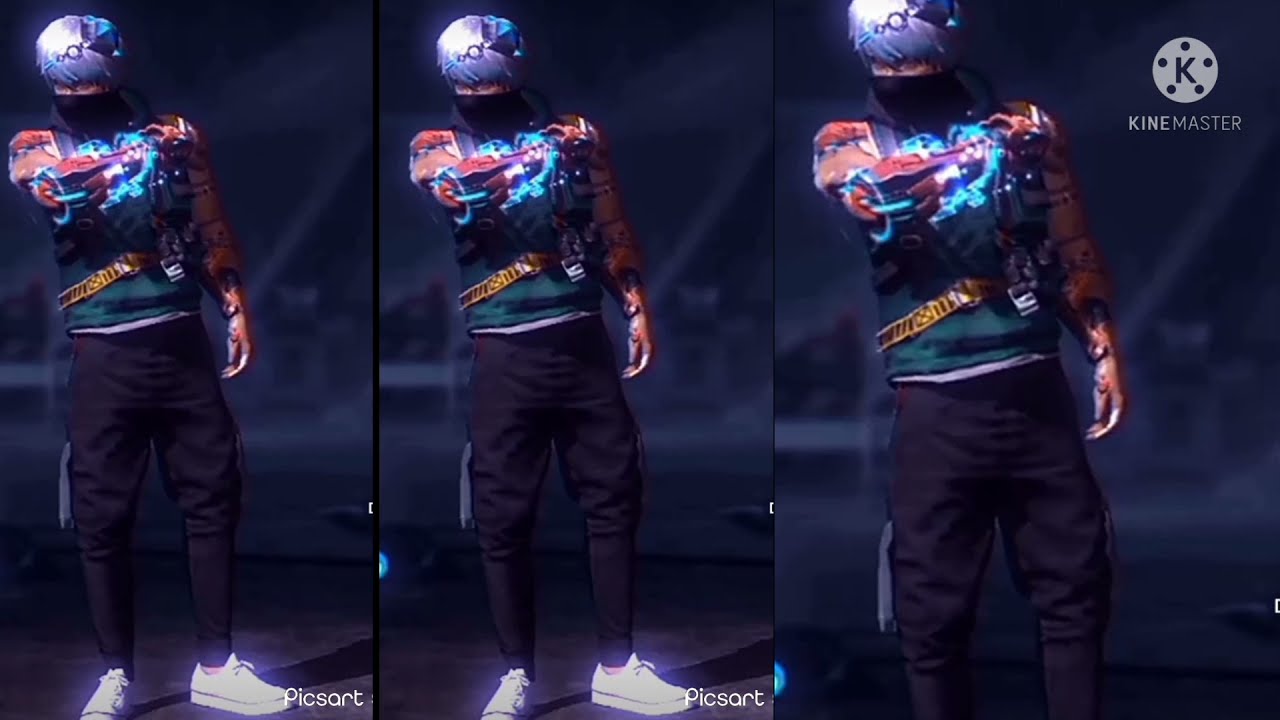The image features a highly detailed, digital illustration of what appears to be a character from a video game or comic book, presented in three repeating panels. The character, a silver-haired young man with light purple tones, wears a face mask and exudes a blend of anime and futuristic aesthetics. Labeled "Pixar" on two panels and "KineMaster" with a distinct K logo in a circle with five dots on the third, the overall scene is set against a stark black background.

The character is dressed in black pants and white sneakers, with additional accessories that include baggy black jeans or cargo shorts with a gray rag. He sports a green shirt under a jacket, enhancing his intergalactic warrior look. Notably, his arms are cybernetic with mechanical, orange-toned limbs, one of which is enhanced with vivid blue electrical energy. The robotic and armored design elements, along with what seems to be an intergalactic gun on his left hand, give the character a tough, battle-ready appearance suitable for the dynamic world of video games or graphic novels.